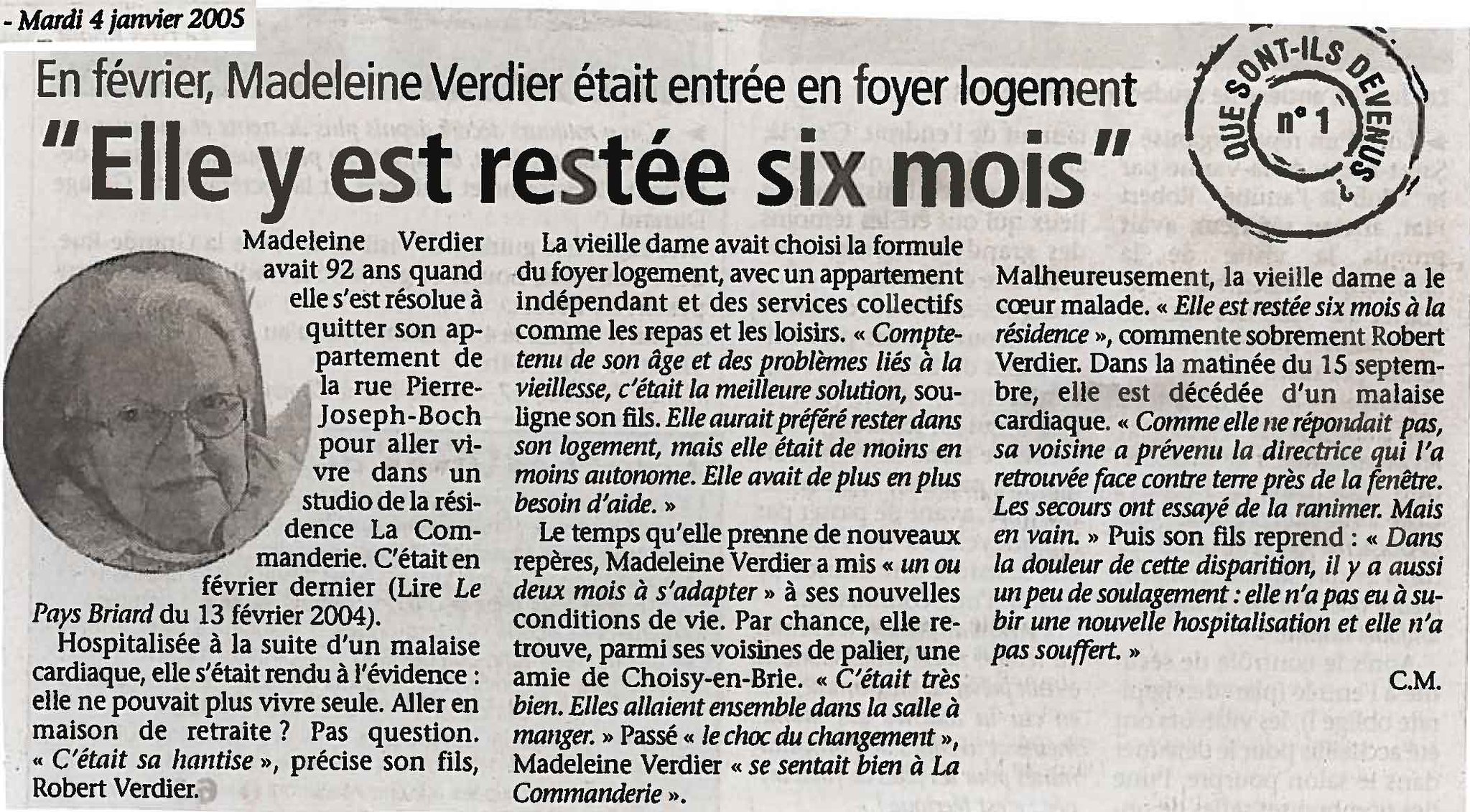This is an up-close photograph of a black-and-white newspaper article, possibly an obituary, written in Spanish. The article is rectangular with a white background and black text. In the upper left-hand corner, there is a date that reads "January 4, 2005," suggesting when the article was published. In the upper right-hand corner, a black circular design contains a smaller circle, with text wrapped around the space in between. Further down, there is an oval photograph of an elderly woman with short gray hair and glasses, wearing a shirt with a visible collar. Her name appears to be Madeline, likely Madeline Verdier, as seen at the beginning of the article. The layout includes three columns of text wrapping around the photograph, detailing some part of her story or life. At the bottom right-hand corner, the initials "C. M." are noted, possibly indicating the author or an editor.